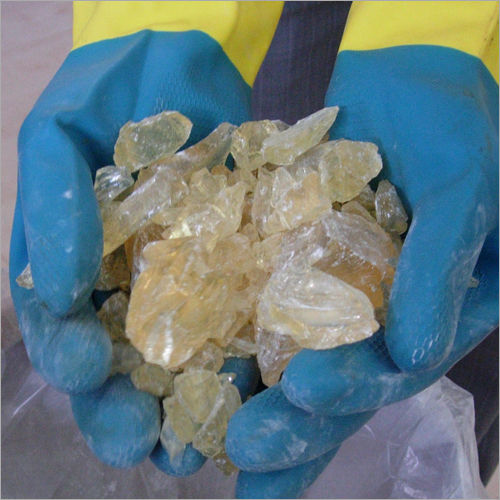The photograph captures a pair of hands, dressed in blue rubber gloves with yellow wrist cuffs, holding a collection of translucent, glossy crystals. The hands, cupped together, present these crystals which vary in size from small fragments to larger chunks. The crystals are primarily clear but display shades of white, yellow, and gold, with a glass-like texture that reflects light. These hands are positioned above an opened, clear plastic bag, partially visible at the bottom of the image. The background features a grayish hue, suggesting a neutral or industrial setting. The scene hints at a careful handling of the crystals, possibly in a controlled environment, like a scientific or archaeological operation.